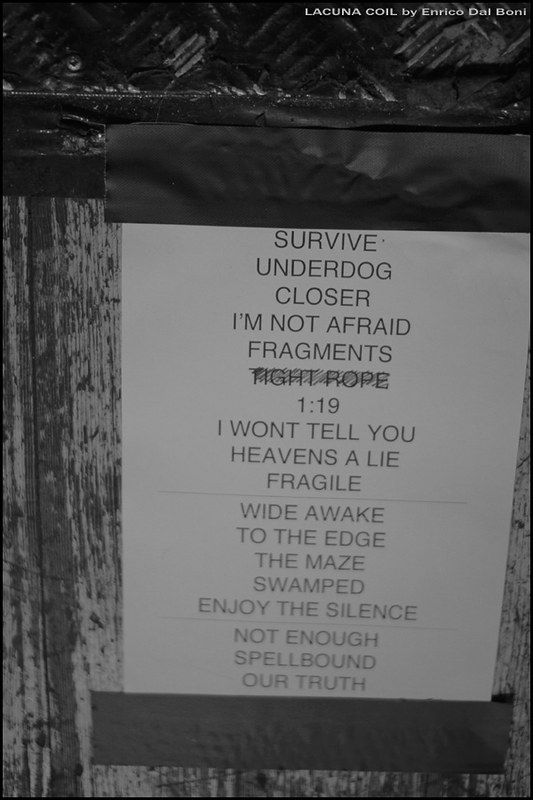The black-and-white photograph, presented in portrait orientation, features a detailed vertical sign affixed to a wooden background with dark tape along the top and bottom edges. This sign, covered in black text written in all caps, lists a series of evocative words and phrases on separate lines: "Survive, Underdog, Closer, I am not afraid, Fragments, Tight rope (with a diagonal strike-through), 1:19, I won't tell you, Heaven's a lie, Fragile, Wide awake, To the edge, The maze, Swamped, Enjoy the silence, Not enough, Spellbound, Our truth." At the top right of the image, nearly hidden in a dark area, delicate white text reads, "Lacuna Coil by Enrico Daltoni," adding a subtle, yet distinctive credit to the photograph. The wooden paneling and the realism of the black-and-white style contribute to the overall striking, gritty aesthetic of the image.